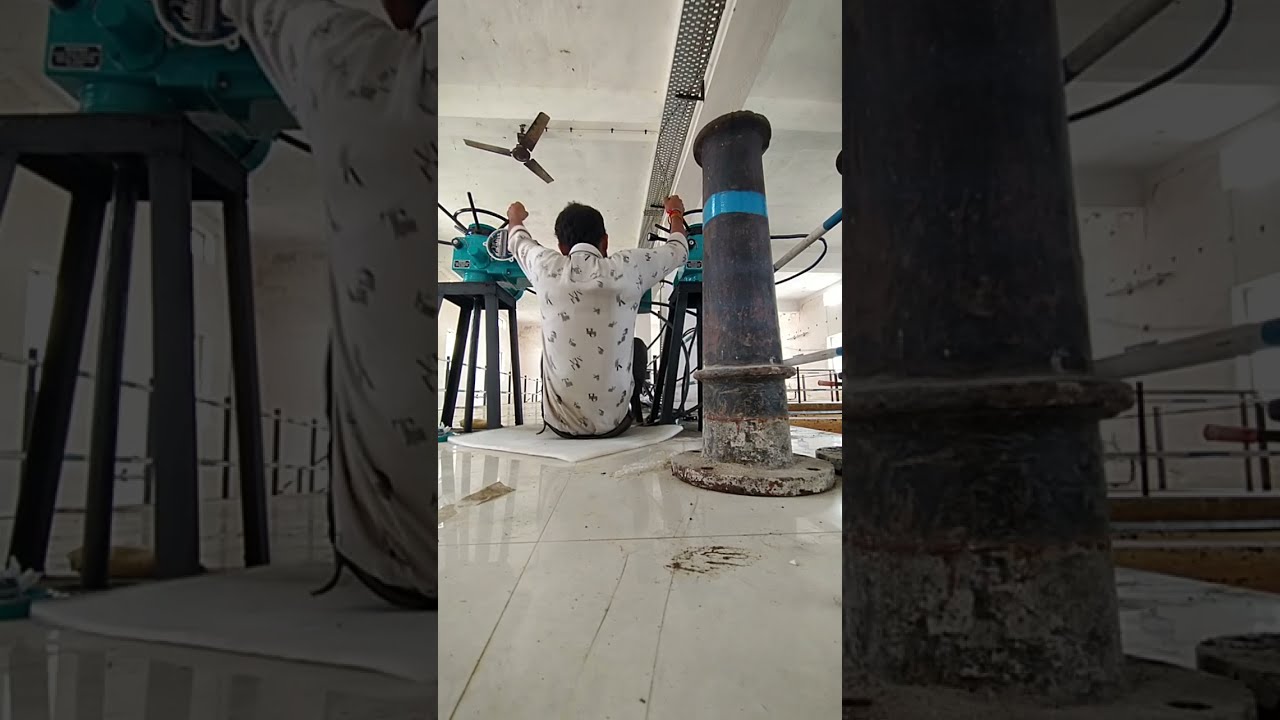This photograph, likely screenshotted from a video or social media reel, captures a man sitting cross-legged on a thin padding in the center of a tiled floor, brightly reflecting the furniture around. His white long-sleeve shirt, speckled with a navy blue pattern, stands out as he works on two identical blue devices with wheels or handles positioned on black stools beside him. The man, seen from behind, appears to be adjusting these mechanisms. The scene, possibly set in a warehouse or factory, features additional elements such as a brown or black ceiling fan to the top left, a large metal pillar resembling a smokestack or ship anchor to his right, and a perforated silver grate on the white ceiling punctuated with various railings and pipes. Natural light fills the room, enhancing the image's clarity.